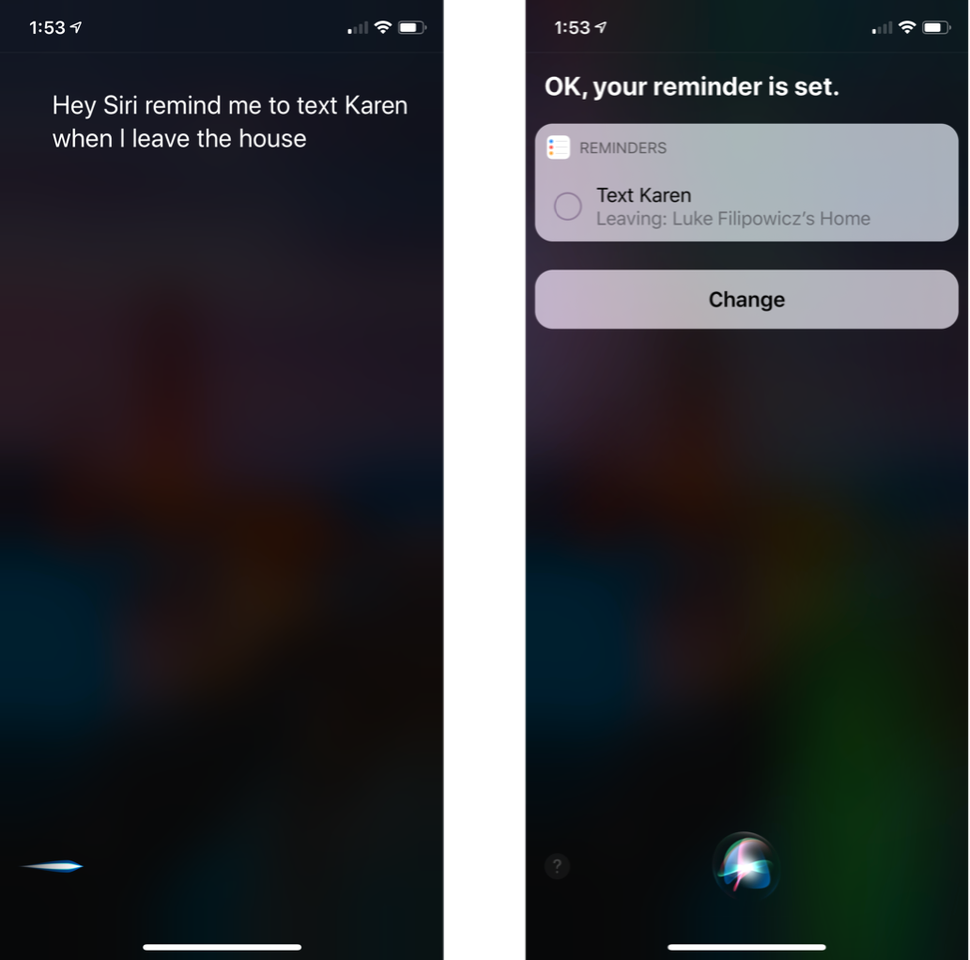**Image Description:**

*The image is composed of two vertical rectangular sections of equal size. The left section displays a mobile device screenshot containing a Siri command, while the right section shows a subsequent confirmation screen.*

**Left Section:**
- **Top Left Corner:**
  - *Time Display:* 1:53
  - *Diagonal Triangle:* A white icon pointing upwards to the right, indicating perhaps an alert or notification.
- **Top Middle:**
  - *Voice Command Text:* "Hey Siri, remind me to text Karen when I leave the house," displayed in white text.
- **Top Right Corner:**
  - *Battery Icon:* Approximately 80% full, indicated in white.
  - *Wi-Fi Signal Icon:* Completely full, suggesting strong connectivity.
  - *Phone Signal Icon:* Only one bar, denoting weak signal strength.
- **Bottom Section:**
  - *White Rectangular Bar:* Positioned at the bottom.
  - *Light Sweep:* Extending from the bottom left across the bottom edge.

**Right Section:**
- **Top Left Corner:**
  - *Time Display:* 1:53 (identical to the left section).
  - *Diagonal Triangle:* The same white icon as seen on the left side.
- **Top Middle:**
  - *Confirmation Text:* "Okay, your reminder is set," displayed in white text.
- **Below Confirmation Text:**
  - *Notification Box:* A rectangular box labeled "Reminders."
  - *Reminder Details:* Includes the task "Text Karen" and the trigger location "Leaving Luke Blupuk's Home."

The overall context of the dual images shows the process of setting a reminder via Siri, first by giving a voice command and then receiving a confirmation.